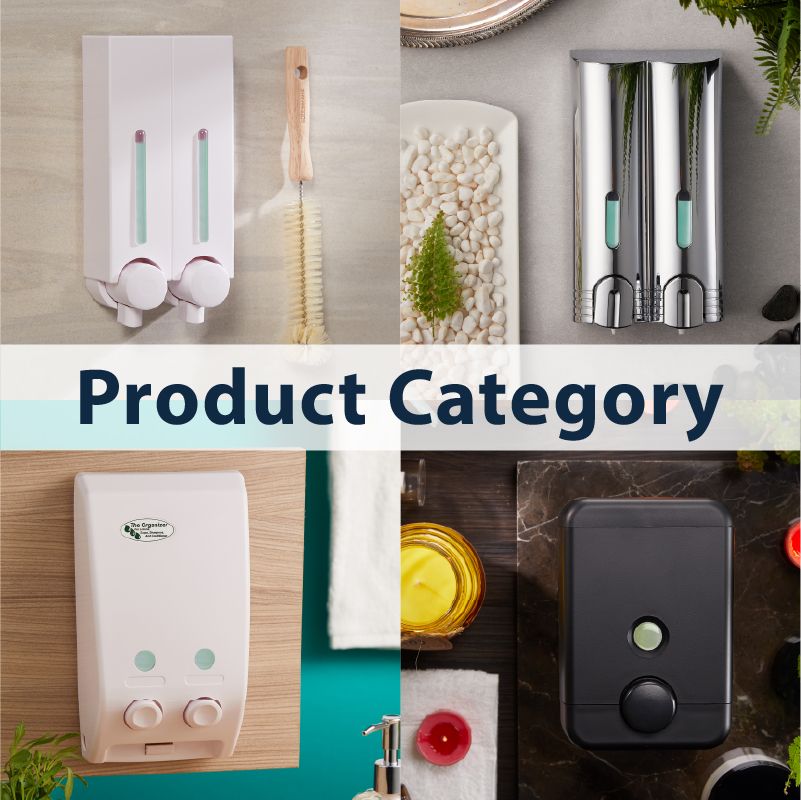This image is divided into four distinct panels with a central bar labeled "Product Category" in blue and white text. The top-left panel displays a white, wall-mounted apparatus featuring two knobs, along with a wooden-handled bristle brush. Adjacent in the top-right panel, a similar silver apparatus can be seen, with part of its fluid level visible through a small window. This panel also features a white tray filled with small white pebbles and a miniature Christmas tree, set against a gray surface with greenery in the background. The bottom-left panel shows a white soap dispenser labeled "Organizer," and a white towel in close proximity. In the bottom-right panel, we see a black soap dispenser surrounded by a yellow candle and a couple of red candles, all placed on a marble surface.